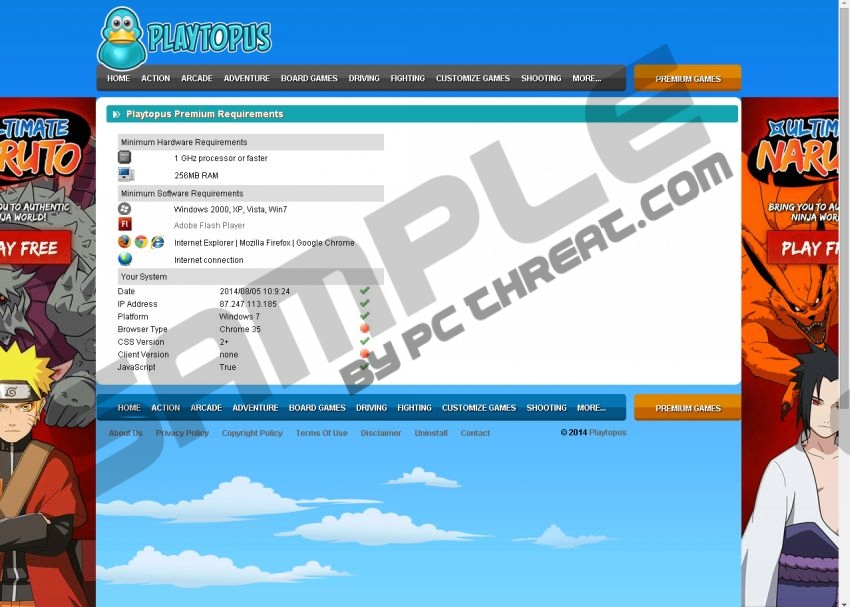This detailed screenshot from the Playtopus website features a comprehensive layout with essential software and hardware requirements. In the top left corner, the distinctive Playtopus logo—a blue duck with a yellow bill—accompanies the website name. Centrally positioned at the top is a menu titled "Playtopus Premium Requirements," leading the content structure.

Beneath this title, the section "Minimum Hardware Requirements" outlines the necessary technical specifications: a processor of 1GHz or faster, and at least 256MB of RAM. Further below, the "Minimum Software Requirements" specifies supported operating systems, which include Windows 2000, XP, Vista, and Windows 7, as well as the essential Adobe Flash Player. Browsers such as Internet Explorer, Mozilla Firefox, and Google Chrome are also supported, along with the necessity for an internet connection.

For user transparency, the section provides an assortment of data about the user's system, listing information such as the current date, IP address, platform, browser type, CSS version, client version, and JavaScript—sourced as a sample by PCthreat.com.

The visual appeal of the screenshot is enhanced by an animation of a cloudy blue sky positioned at the bottom center, adding a dynamic element to the otherwise static page. Flanking this animation on both sides are ads for Ultimate Naruto, featuring anime-style artwork and inviting users to "Play Free."